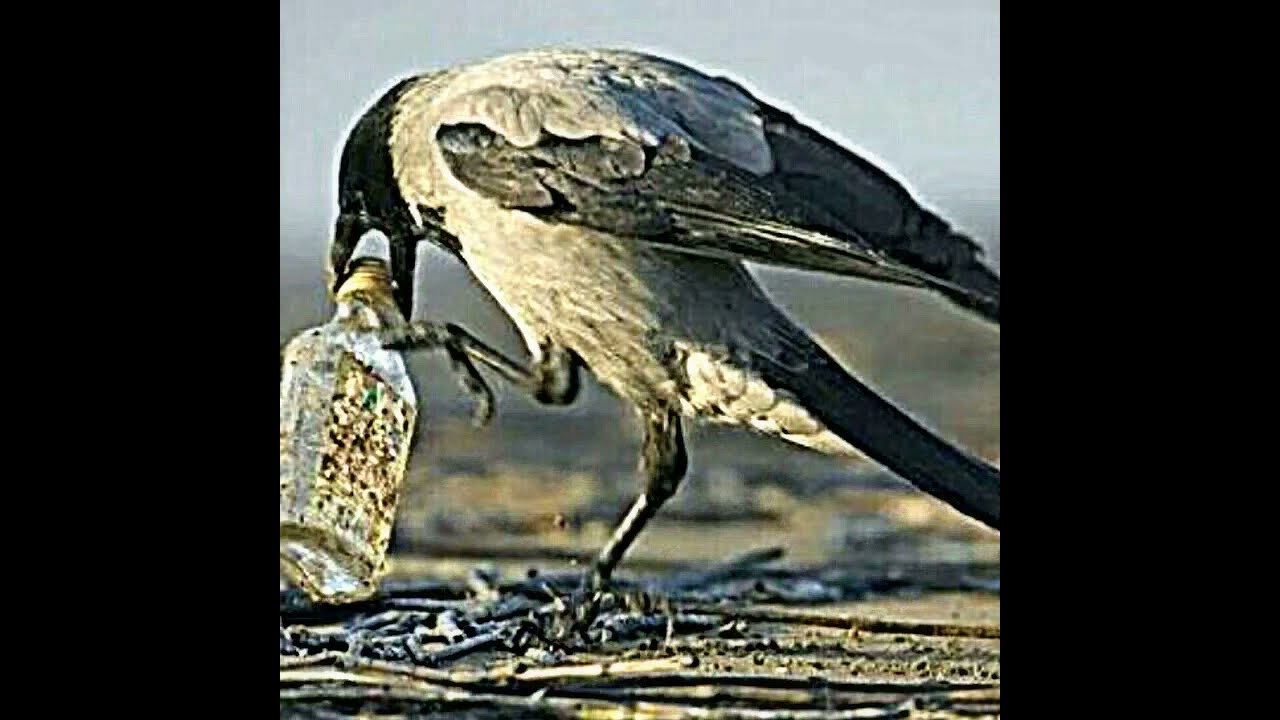This is an older, hazy, and grainy photograph of a bird with distinct black and white plumage, captured in an outdoor setting. The black-beaked bird, featuring a black head, white body, and black wings, legs, and feet, is engaged in an unusual activity—it is trying to twist off the cap of an empty glass bottle that resembles a whiskey bottle. The bird uses its long black beak to grip the lid, while its right foot rests atop the bottle and its left foot remains firmly planted on the dry, sandy ground strewn with thin sticks and branches. The setting is blurred, with a blue and hazy sky in the backdrop. The bottle, adorned with a faded and dirty label, is clutched tightly by the bird, whose determined posture dominates the center of the image. The photograph excellently captures a rare and candid moment in nature.